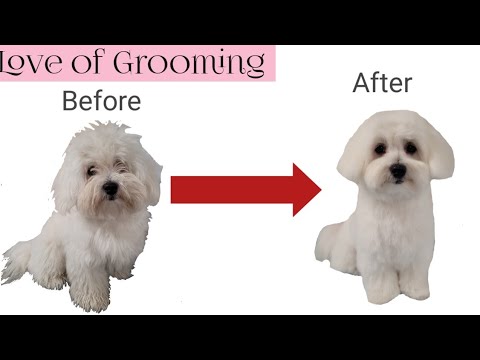The image is an advertisement for a dog collar, featuring a detailed before-and-after grooming transformation of a small white dog. In the "before" picture, the dog appears scruffy, with overgrown fur covering its eyes, dirty fur around its feet, and an untrimmed tail. The "after" picture shows the same dog, now neatly groomed, with trimmed ears, feet, and tail, and its fur clean and white. A red arrow points from the "before" picture to the "after" picture, emphasizing the dramatic change. The words "Before" and "After" are displayed above each respective image in black font. The advertisement's tagline, "Love of Grooming," is prominently featured in the top left-hand corner within a pink text box, with black lettering. The entire image is framed by two black bars, one at the top and one at the bottom, against a white background.